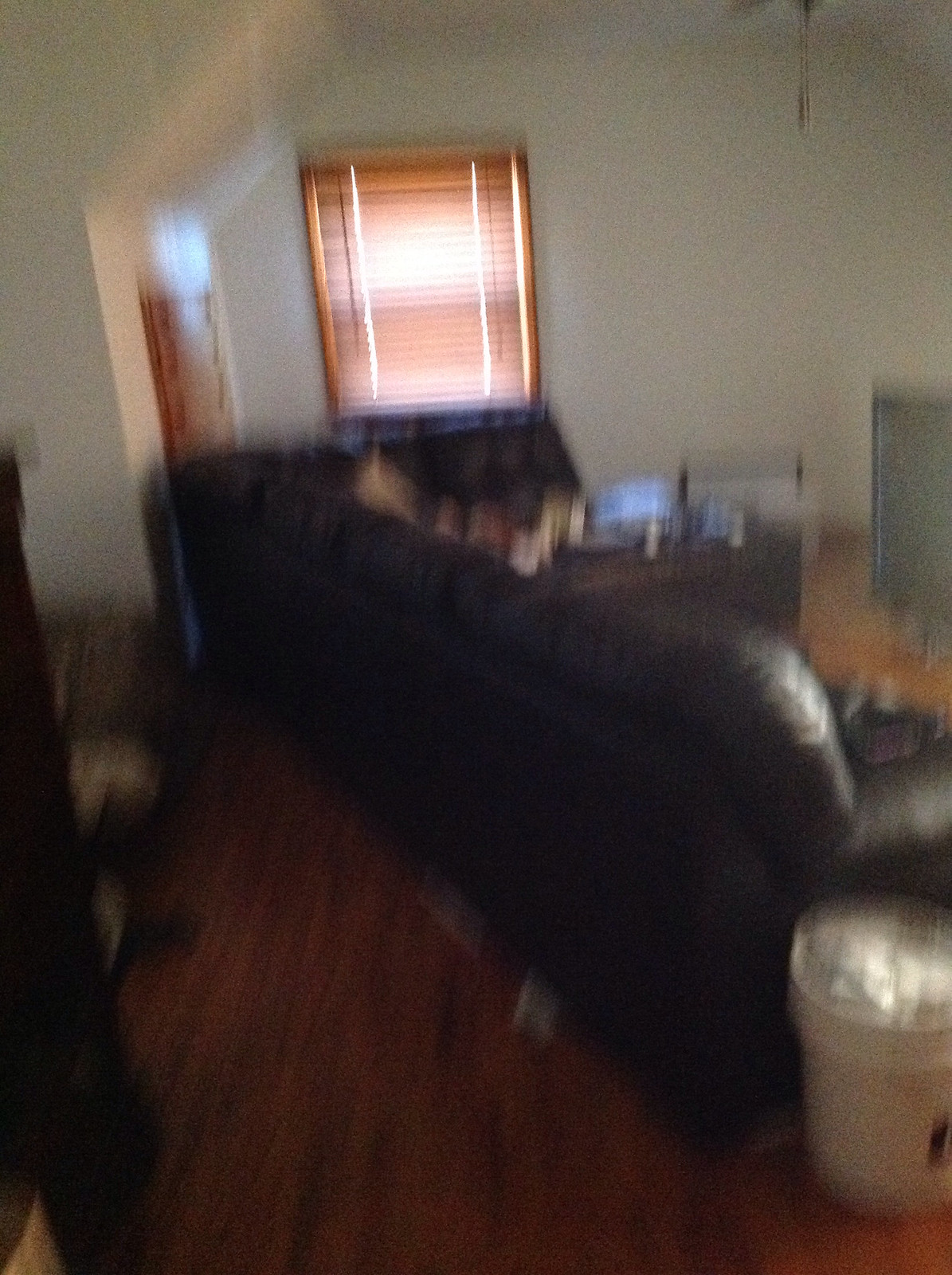This indoor photograph depicts a dimly-lit living room, taken from an unclear angle, resulting in excessive blurriness. The illumination primarily emanates from two windows; the first on the right side of the room, casting reflections onto a dark leather sectional sofa or chair, and the second directly ahead, fitted with closed brown blinds that appear to have a wood-like texture. The walls are painted white, and there's a hint of a doorway visible in the background. The floor is a rich, dark wood or laminate, contributing to the room's cozy yet understated ambiance. On the floor to the bottom right, a white bucket containing what seems to be plastic items can be seen. Meanwhile, an indistinct piece of furniture or object occupies the bottom left corner of the photograph. Overall, the image fails to capture sharp details due to its poor focus but attempts to portray a comfortable and organized living space.